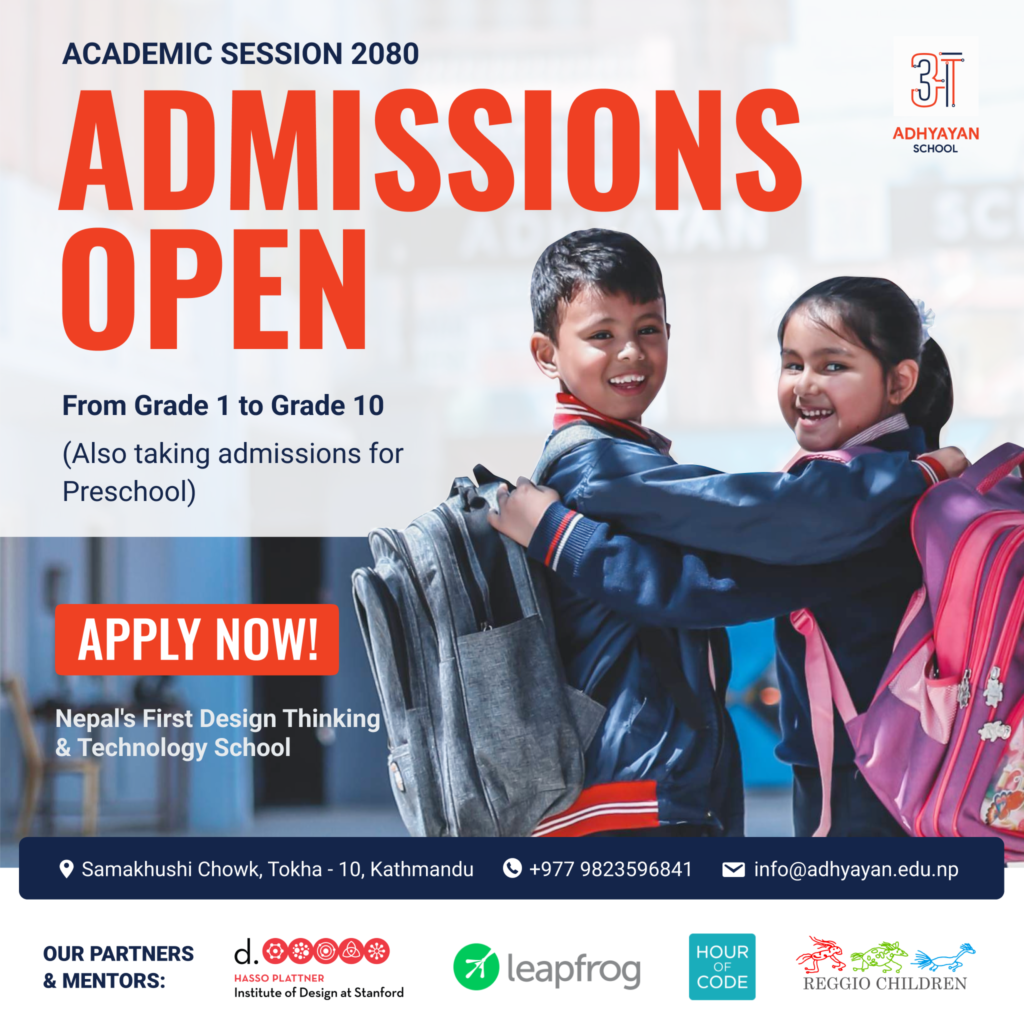The vibrant poster features a heartwarming image of two children embracing. The boy on the left sports a gray backpack, while the girl on the right carries a purple and pink backpack. Both children are dressed in matching blue sweaters adorned with red stripes on the sleeves and hem. 

The poster’s text is artfully displayed in a combination of red, black, and white. In the upper left corner, "Academic Session 2018" is written in black. Below this, the phrase "Admissions Open" is prominently highlighted in bold red letters. Further down in black text, it states, "From Grade One to Grade 10" and additionally mentions the availability of preschool admissions. The bottom of the poster features a call to action in white text on a red rectangular background, urging viewers to "Apply Now."